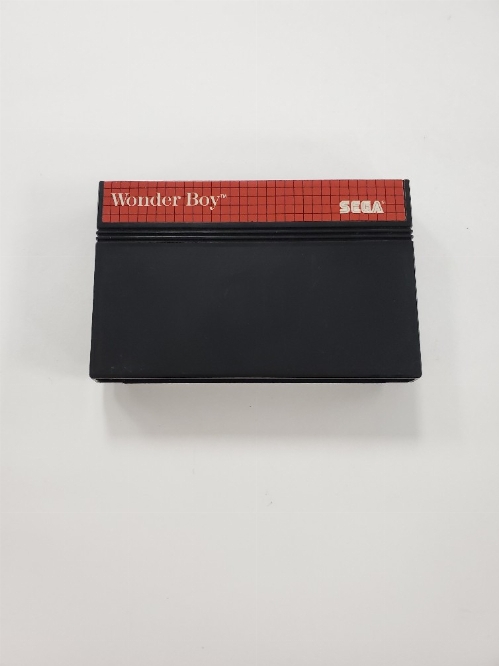This is a color photograph in portrait orientation featuring an old video game cartridge, identified specifically as a "Wonder Boy" cartridge from SEGA. The cartridge is rectangular and predominantly black, positioned slightly above the center of the image, more toward the top, against a solid light gray background. The top of the cartridge displays a red strip with a black checkerboard pattern on the left margin. Centrally placed within the red strip is the title "Wonder Boy" in white text, while the bottom right corner features the SEGA logo, also in white. The image captures a slight shadow beneath the cartridge, adding depth to the scene. The overall style of the photograph is representational realism, focusing on the nostalgic and collectible nature of the gaming cartridge.